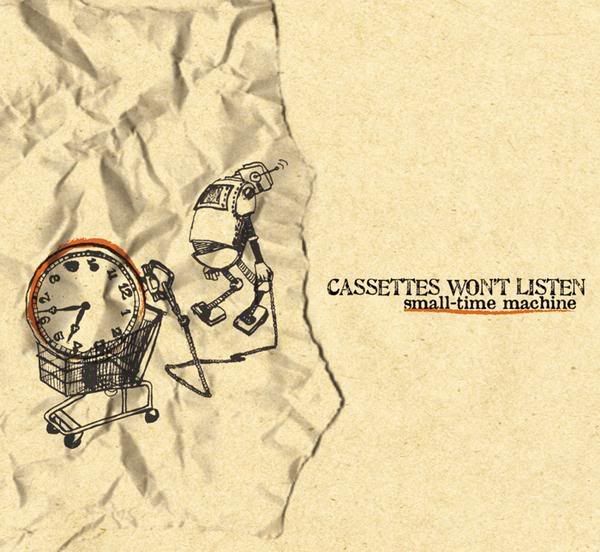The image features an artsy, beige-toned background with a prominent, black-outlined robot walking on the left side, holding a device that leaves marks on the ground. The robot seems to be tethered by a rope to a shopping cart containing a clock, encircled by an orange ring. The scene includes a crumpled paper texture, providing a unique, textured artistic style. Elements such as white circles and various line objects are scattered, enhancing the intricate design. In the foreground, faint white text reads "protect more of your memories for less" above a white bar, while bold black letters state "Cassettes Won't Listen, Small Time Machine," suggesting this might be an album cover or promotional artwork for a music artist. The overall composition, accented with occasional red highlights, positions most elements toward the left, with the text subtly distinct to the right.